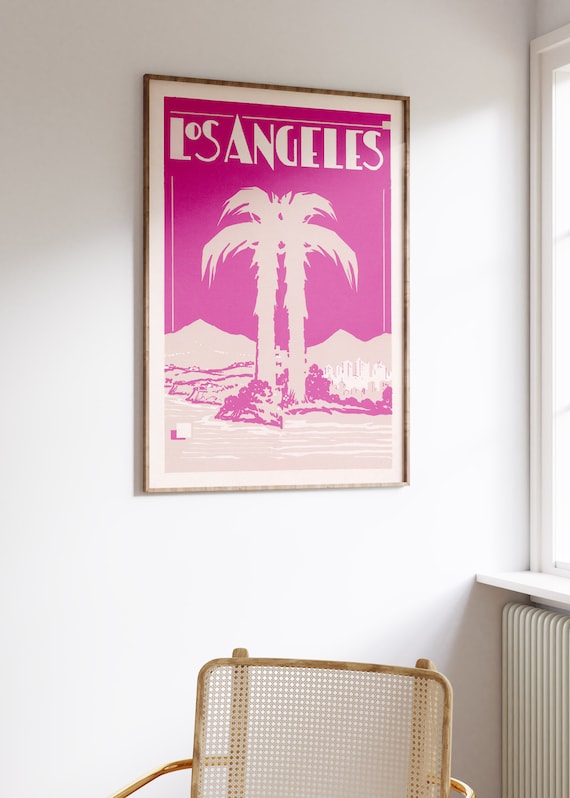The color photograph captures the corner of a white-walled room illuminated by bright sunlight streaming through a window on the right. The window, encased in a white frame with a white flat sill, sits above a white metal radiator. A light tan chair with a wicker backing and thin wood frame is positioned below the window's ledge. The focal point of the image is a wall hanging mounted on the white-painted wall to the left. The hanging features a poster with a light brown wood frame and a wide white border, showcasing a scene with a bright pink sky, gray ground, and two white palm trees. In bold white letters, the poster reads "Los Angeles," with mountains in the background and hints of cityscape on the right. The vibrant pink of the poster contrasts sharply with the predominantly white room, making the artwork stand out.